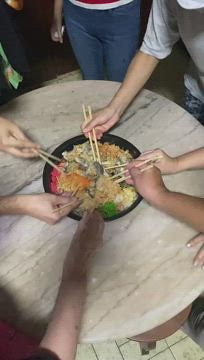This is a low-resolution color photograph capturing a communal meal shared by six people, each visible through their reaching right hands holding light brown wooden chopsticks. The group surrounds a small, round table crafted from light wood with distinct beam-like grain patterns, situated on yellow tiled flooring. At the center of this intimate scene is a large black bowl, brimming with a colorful mix of rice, noodles, vegetables, and meat featuring shades of yellow, green, and light red. The image primarily focuses on the arms extending towards the shared dish, but towards the top, the bottom of a woman’s jeans and an elbow-length blouse can be seen, adding a subtle hint of the diners' attire.